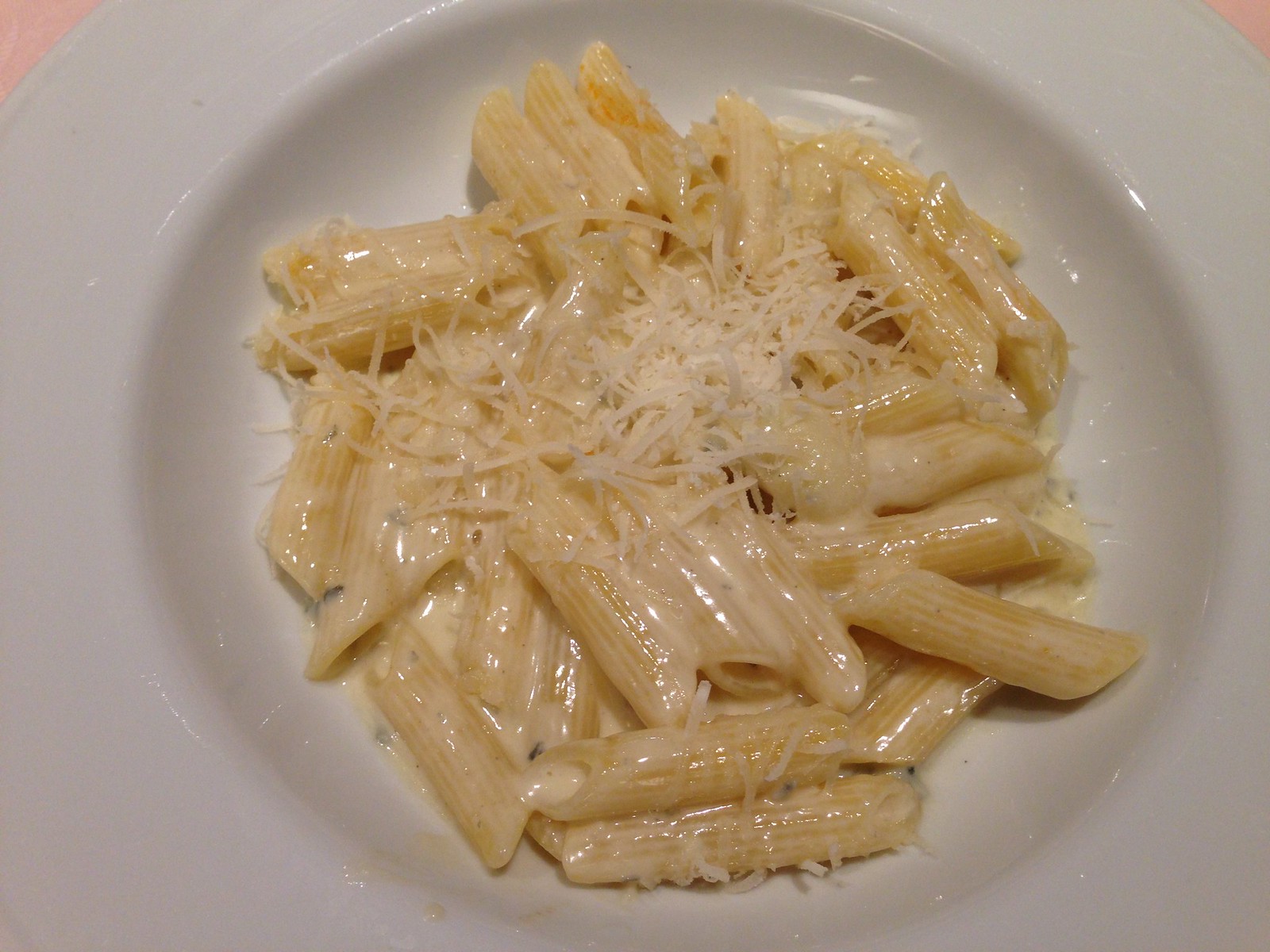This indoor photograph, styled with a focus on a single object, presents a close-up, top-down view of a small ceramic bowl of penne pasta smothered in a creamy, yellow cheese sauce. The penne, characterized by its distinctive striations, glistens under the light, highlighting the gooey cheese and the generous sprinkling of grated cheese, probably mozzarella or parmesan, on top. The shiny, white bowl, slightly reflective due to the camera flash, gives a hint of the table's pink hue at the top corners, suggesting a restaurant setting. The bowl appears to be a deep, ceramic dish, containing a modest, single-serving portion of the cheesy pasta.